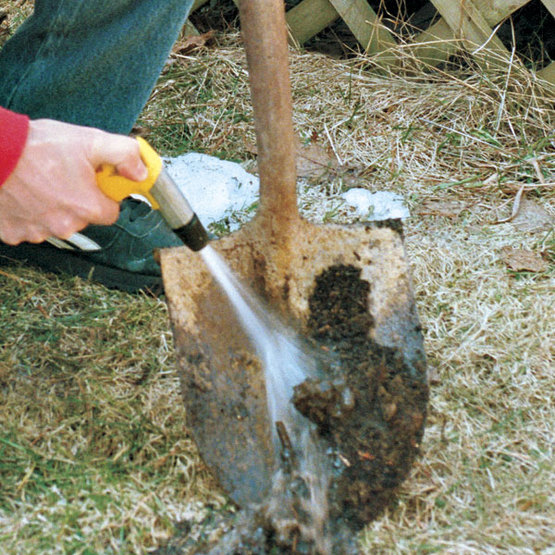The image portrays a close-up scene of an individual in a red shirt, blue jeans, and athletic shoes, using a yellow-handled, silver nozzle with a black tip to spray water and clean a dirt-covered, rusted spade shovel. The spade, resting on green grass amidst a straw-like area, appears to have been used for shoveling dirt or manure. In the background, a latticework fence adds a crisscross pattern to the scene, suggesting an outdoor, possibly agricultural or gardening setting. The person is actively squeezing the nozzle to wash off the shovel, indicating a vigorous cleaning process.